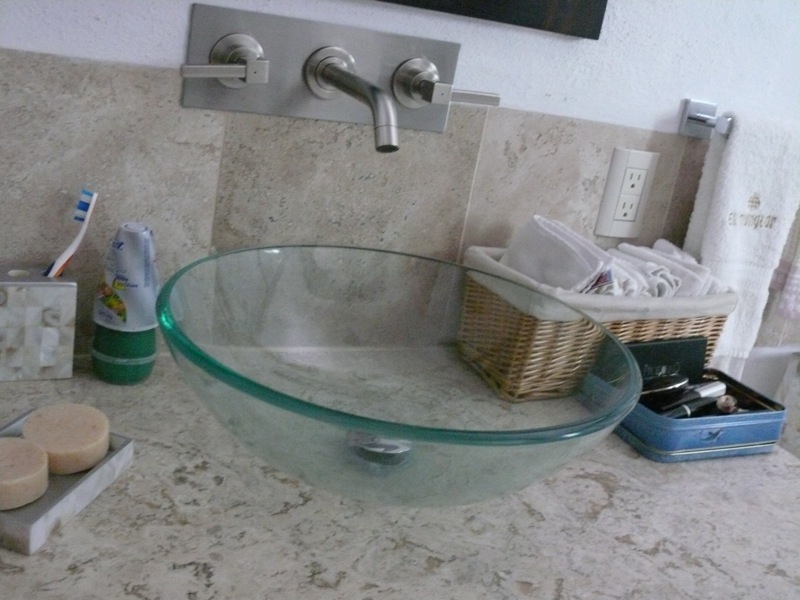The image showcases a meticulously designed modern bathroom characterized by its sleek, built-in fixtures and contemporary elements. The wall, adorned with large brown-tan and white tiles, serves as a backdrop for two minimalist taps and a wall-mounted faucet, seamlessly integrated without visible piping. Four tiles are visible in the frame, each contributing to the elegant aesthetic.

Above the fourth tile, from left to right, is a stylish towel rack holding a pristine white towel adorned with unreadable gold writing. Adjacent to the towel rack is a convenient outlet. A cleverly repurposed bread basket, lined in cream fabric, sits on the countertop, filled with neatly folded washcloths. In front of this basket rests a blue tin container, holding various makeup items, including a tube of lipstick and a makeup brush.

A striking feature of the countertop is a large, green glass bowl sink, complete with a central drainage hole. Next to this is a green Glade air freshener, adding a touch of freshness to the space. A mosaic-tiled toothbrush holder stands nearby, holding a toothbrush with blue and white bristles, alongside an orange and blue handle. Completing the arrangement is a stone soap dish, characterized by its grayish tone and brown veining, containing two round disc soaps.

This modern bathroom's design is both functional and artistic, reflecting a keen attention to detail and a blend of practicality with aesthetic appeal.